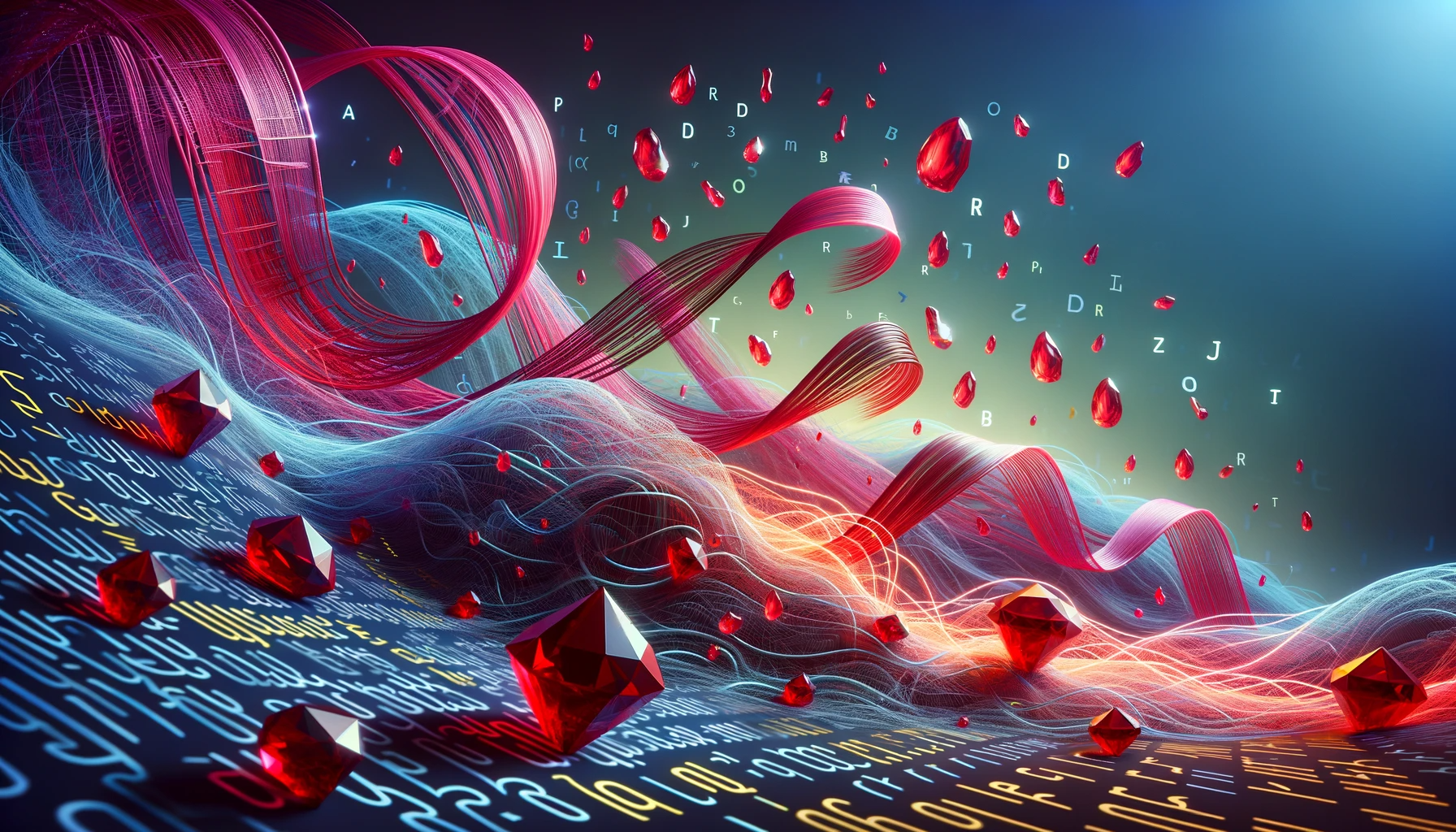The image is a highly detailed, AI-generated artwork featuring a rich tapestry of vibrant elements. The background is primarily dark blue with light radiating from the top right corner, creating a luminous effect. The scene is divided diagonally by a series of multicolored, ribbon-like lines, splitting the image into two contrasting halves. 

In the upper portion, ruby gemstones of various shapes—some fully faceted, others partially—float amidst randomly scattered alphabet letters. These letters, along with the rubies, dance in the sky-like background. The lower portion transitions into a ground-like surface, decorated with more ruby gems interspersed among wavy ribbons of blue, orange, and pink, which resemble flowing spaghetti. The bottom left is especially filled with a field of text and symbols, including yellow and blue shapes that hint at letters but are more abstract. The overall composition of the image conveys a sense of dynamic movement and a fusion of natural and digital aesthetics.